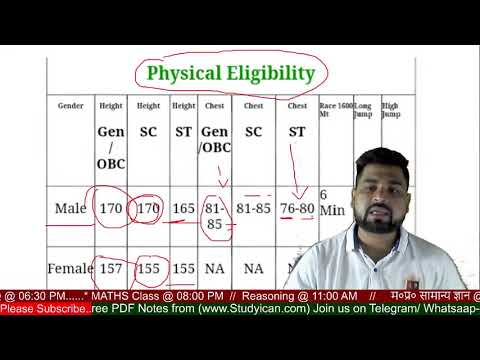The image appears to be a screenshot of a video or show, featuring a darker-skinned man in the lower right-hand corner. The man has short black hair, a black beard, and is wearing a white polo shirt with a red logo on the left side for the viewer. He seems to be speaking as his mouth is open. Behind the man, there is a white screen displaying a chart and the heading "Physical Eligibility" written in green, highlighted by a red circle. The chart includes columns labeled "Gender," "Height," "Chest," "Race," "Long Jump," and "High Jump," with rows underneath listing "Male" and "Female" followed by various numbers. Along the bottom of the screen, there is informational text including a dark red banner with white lettering and a red square that says "Please Subscribe," as well as a dark green banner with additional information, such as "Maths class at 6:30 p.m.," "Reasoning at 8:00 p.m.," and "PDF notes from studyican.com." The text also mentions joining on Telegram/WhatsApp.